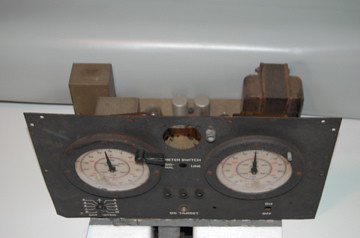This photograph showcases a complex mechanical component fixed on a flat, gray metallic front plate. The front surface, possibly painted, features various knobs and meticulously detailed illustrations and labels scattered across its edges and center. Prominently displayed on the left and right sides are two circular gauges, each with a delicate hand pointing to numerals set against a white background. These gauges are intricately marked with blue and red lines, numbers, and letters, emphasizing their functional elegance.

The entire setup is placed indoors, resting on a pristine white surface with a stark white background. The scene is illuminated by a bright ceiling light, evident from a horizontal reflection line across the backdrop. This sharp lighting highlights the mechanical unit’s features without introducing any external distractions.

Behind the metallic front, the component reveals a more intricate assembly of parts. Central metallic cylinder shapes dominate this rear view, flanked on either side by robust, blocky brown elements. These brown components, appearing as chunks, exhibit a texture and color that could either be of wood or metal, adding to the intrigue of the device's construction.